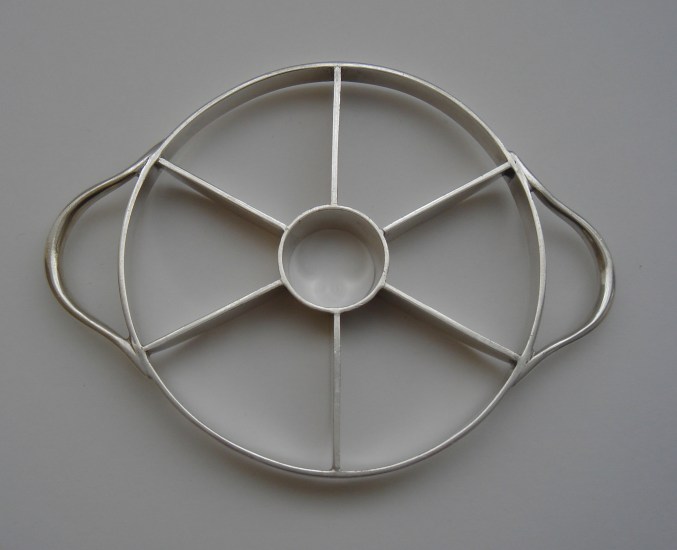The image depicts a metal apple cutter positioned on a light gray, flat surface. The tool is centered in the image, and it is slightly flipped upside down, emphasizing its structure. The apple cutter is circular in shape with a smaller circle in the middle designed to remove the core of the apple. Surrounding the central circle are six triangular cutouts that serve to slice the apple into equal sections when the cutter is pushed downwards. The device includes curved steel handles on the far left and right, which are welded to the outer circle, providing a firm grip during use. The apple cutter's metal construction includes colors of white, silver, and gray, giving it a sleek and durable appearance. The overall setting is well-lit, highlighting the details of the tool and its potential use for efficiently slicing apples.